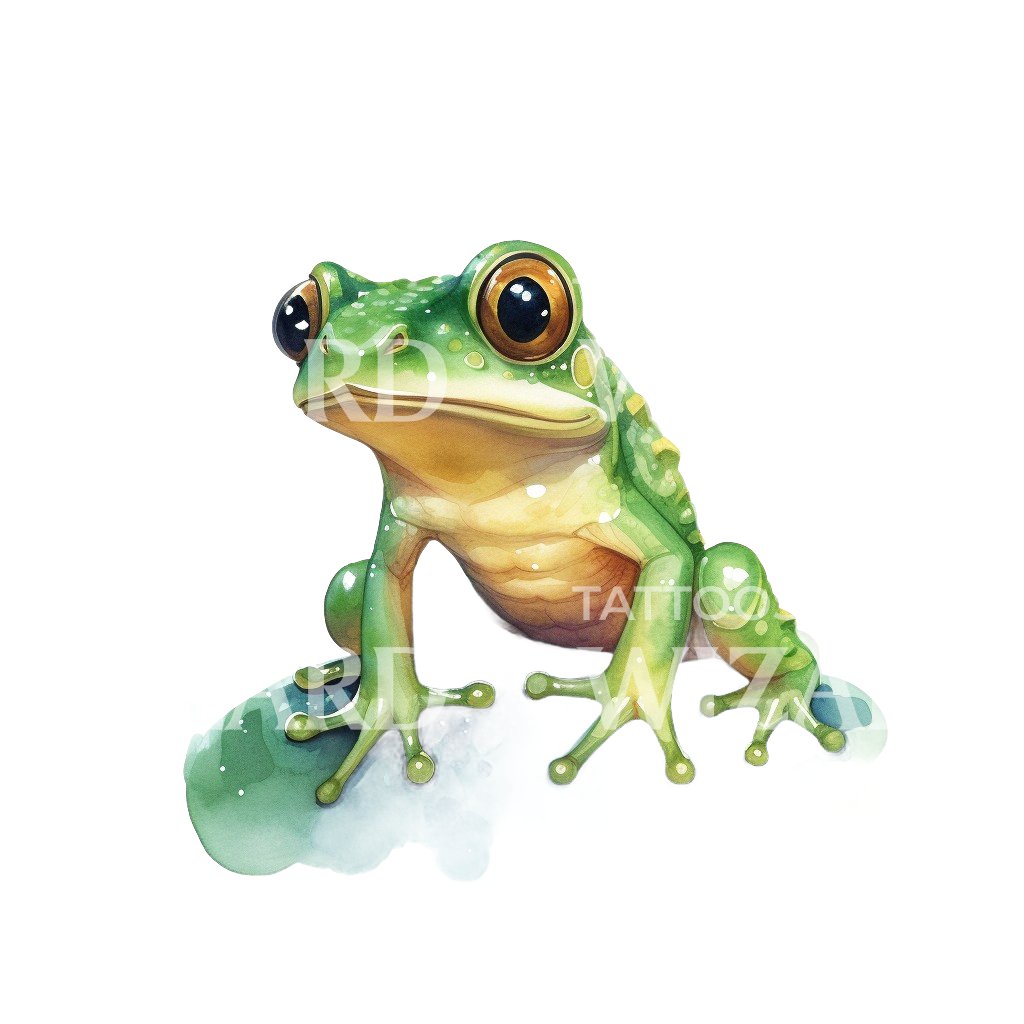This detailed image features a computer-generated illustration of a green frog with large, expressive brown eyes that have black irises dotted with specks of white, reflecting light. The frog is situated against a solid white background with no borders, standing upright and slightly tilted to its right, the viewer's left. Its body is predominantly green and peppered with white and yellow spots, transitioning to a textured tan underside. The frog's limbs are green with tan blending in, with its front legs having four toes each, while the right front leg has three toes. There is an irregularly shaped splotch of green and white or gray paint on the lower left side of the image. Superimposed on the white background is a faint, hard-to-read watermark with the capital letters "RD," the word "tattoo," and the letters "CWZ," which blend into the background and are partially obscured.